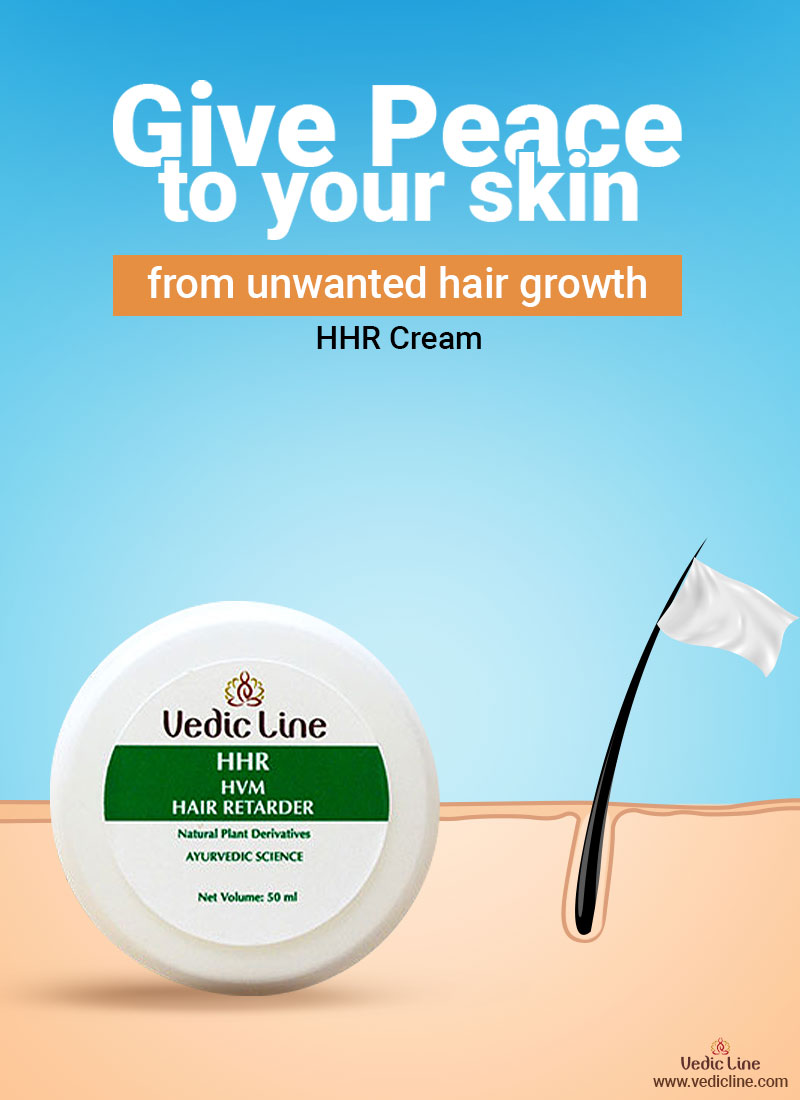The advertisement is a rectangular image taller than it is wide, with a blue gradient background occupying the upper three-fourths, transitioning from a deeper blue at the top to a lighter blue towards the bottom. At the top in bold white sans-serif text, it reads "Give peace to your skin," with "to your skin" slightly overlapping "give peace." Below this phrase, an orange rectangle with white text states "from unwanted hair growth," and beneath this, in black text, it says "HHR cream."

In the lower portion of the image, the background transitions to a light peachy-pink color, resembling magnified skin. On the right side, there is a single strand of black hair emerging from the skin, waving a white flag at its top, symbolizing its surrender. To the left, there is a circular product image with a white label. The label features a black "Vedic Line" logo, a green banner stating "HHR HVM Hair Retarder," and beneath this, green text details the natural plant derivatives, Ayurvedic science, and a net volume of 50 milliliters.

The lower right corner of the image displays the "Vedic Line" logo again in black text, alongside their website URL, www.vedicline.com.